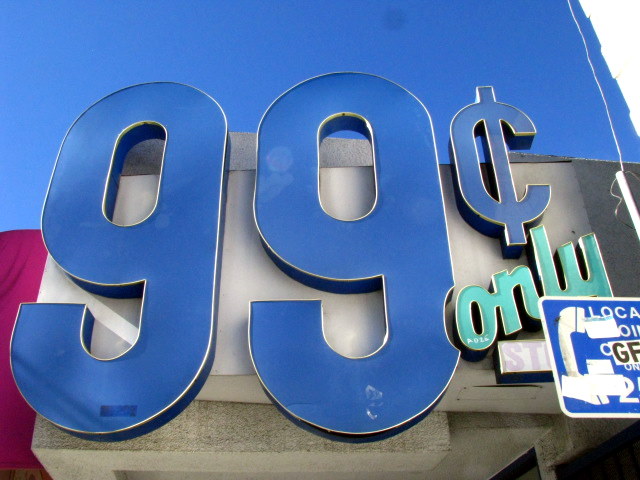This color photograph captures a detailed close-up of a section of a retail store exterior. The prominent metallic sign features large blue numerals "99" and a blue cent symbol attached to a grey concrete wall. Directly beneath the cent symbol, the word "only" is elegantly written in a light green cursive script. The upper portion of the image showcases a bright blue sky. In the bottom right-hand corner of the frame, there's a smaller blue sign with white text that appears to spell out "L-O-C-A." This secondary sign also features a depiction of an old-fashioned rotary phone handset and is partly obscured by a glare. A small white sticker with the black letters "GF" is visible nearby. The lower portion of the image, cast in shadow, reveals more of the concrete structure, which could be the underside of the building's roof, while a narrow rectangle of dark pink is noticeable in the left-hand corner.